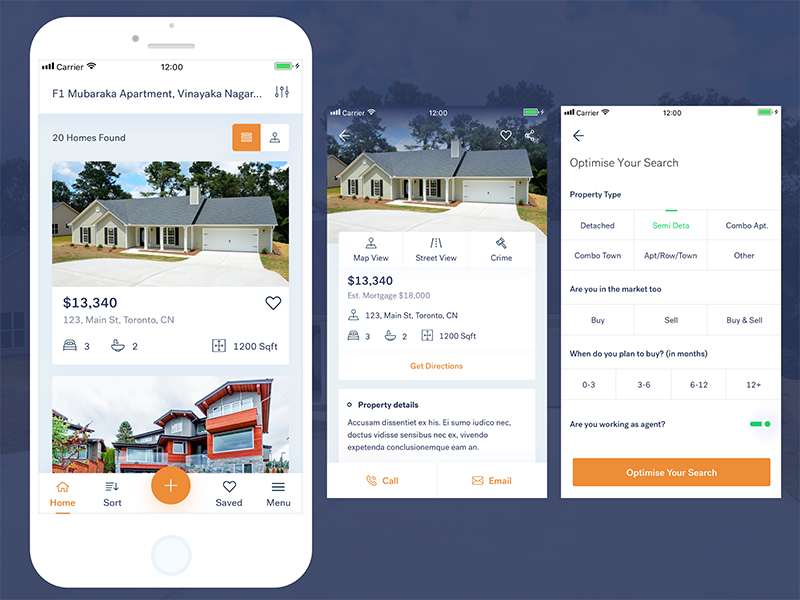The photograph depicts a smartphone screen displaying a real estate app at 12 o'clock, showing a strong carrier signal and nearly full battery indicated by a green icon. The app interface is focused on property listings in F1 Mabarka Apartment, Vinaka, although the city name is partially obscured with ellipses. 

The primary listing features a detailed overview of a ranch house located at 123 Main Street, Toronto, Canada. The property spans 1,200 square feet and is valued at $13,340. Adjacent to this, a smaller thumbnail image of a red, raised house closely situated next to a brown house on the left is visible. The specific details of this second listing are cut off, but control icons for sorting, sharing, and menu options are clearly present at the bottom of the screen, alongside an orange circular "plus" button.

Switching to another view, the app presents a closer image of the initial ranch house, highlighting street view, map view, and crime statistics. The address is reiterated, and the mortgage amount is indicated as approximately $18,000. Property dimensions and features are summarized with 1,200 square feet and icons denoting either two or three unspecified attributes, possibly bedrooms and bathrooms. An orange "Get Directions" button is available, alongside quick links for property details, and options to either call or email the listing agent.

A tertiary image labeled "Optimize Your Search" introduces an interactive interface where users can specify property types, as well as their buying intention (buy or sell) and timeline, ranging from zero to more than five months. An orange bar at the bottom encourages users to optimize their search parameters further.